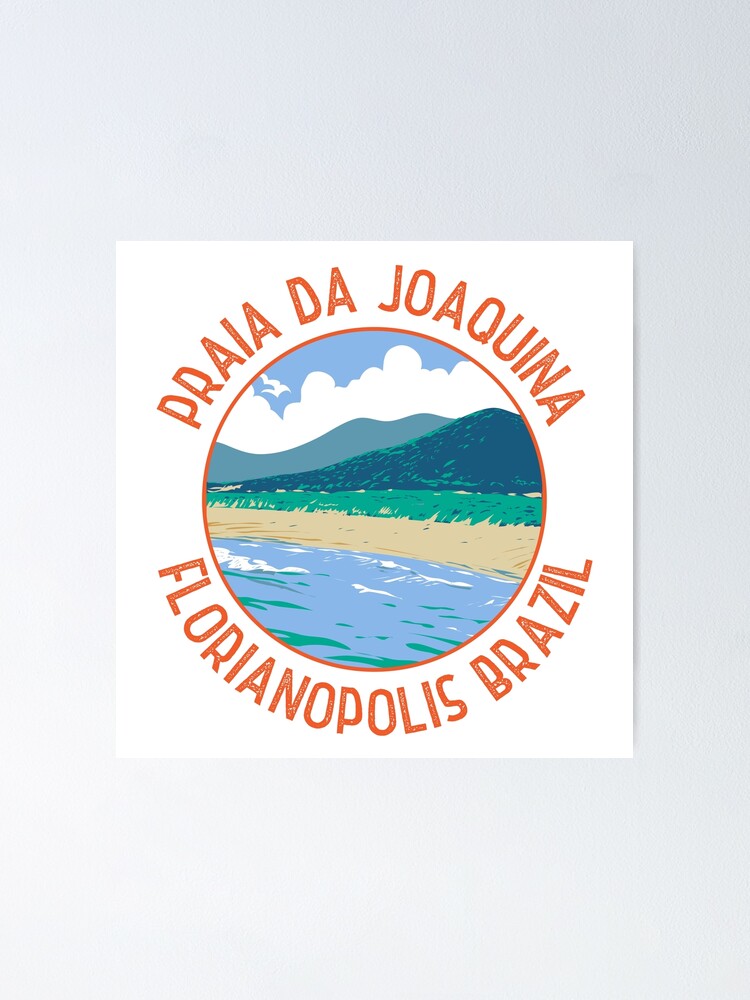The image is a photograph of a square print or sticker placed on a plain white surface. The print features a round illustration bordered by a thin, dark orange band. In dark orange capital letters, the text reads "Praia da Joaquina" at the top and "Florianopolis, Brazil" at the bottom. Inside the circular illustration is a stylized beach scene with blue waves with white foam breakers, followed by a stretch of golden beach. Beyond the beach, there's a rising green landscape that transitions into dark green mountains. The background includes stylized white clouds scattered across a blue sky, creating a picturesque coastal view. Though the illustration is not highly detailed, it effectively captures the essence of the coastline scenery.